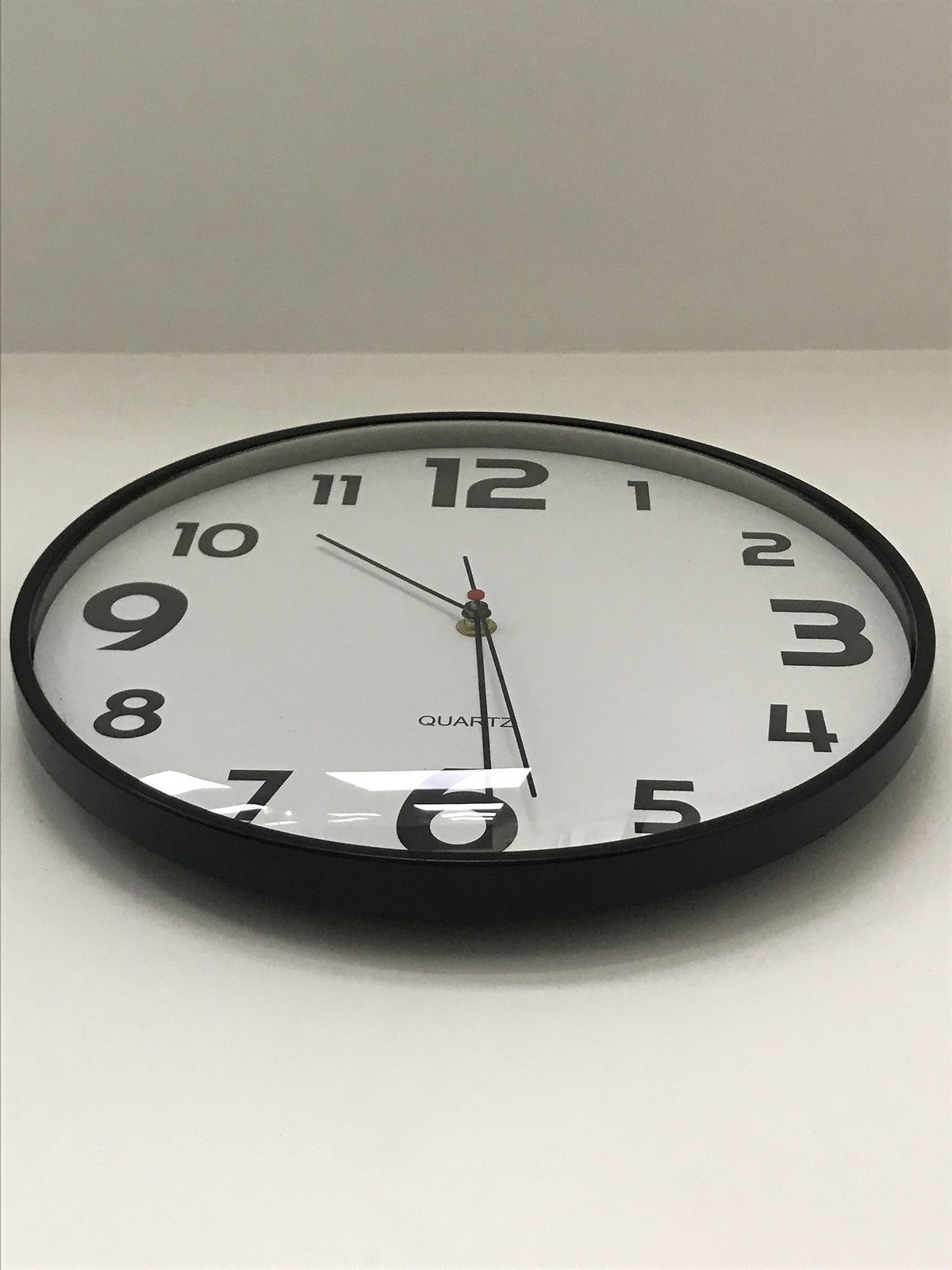The image depicts a large, black-rimmed, circular wall clock, commonly found in places such as schools or doctor's offices. The clock, positioned high on a wall close to the ceiling, casts a dark shadow on the ceiling above. It is an analog clock featuring a white face with bold black numbers, where the 12, 3, 6, and 9 are much larger than the others. The clock displays the time as 10:29, with the minute hand almost at 6, and the hour hand between 10 and 11. The clock also has a very long, thin second hand, which along with the hour and minute hands, revolves around a central pin that is red in color. The clock bears the word "quartz" above the 6, possibly indicating its brand. A layer of glass covers the clock face, reflecting the ceiling lights.